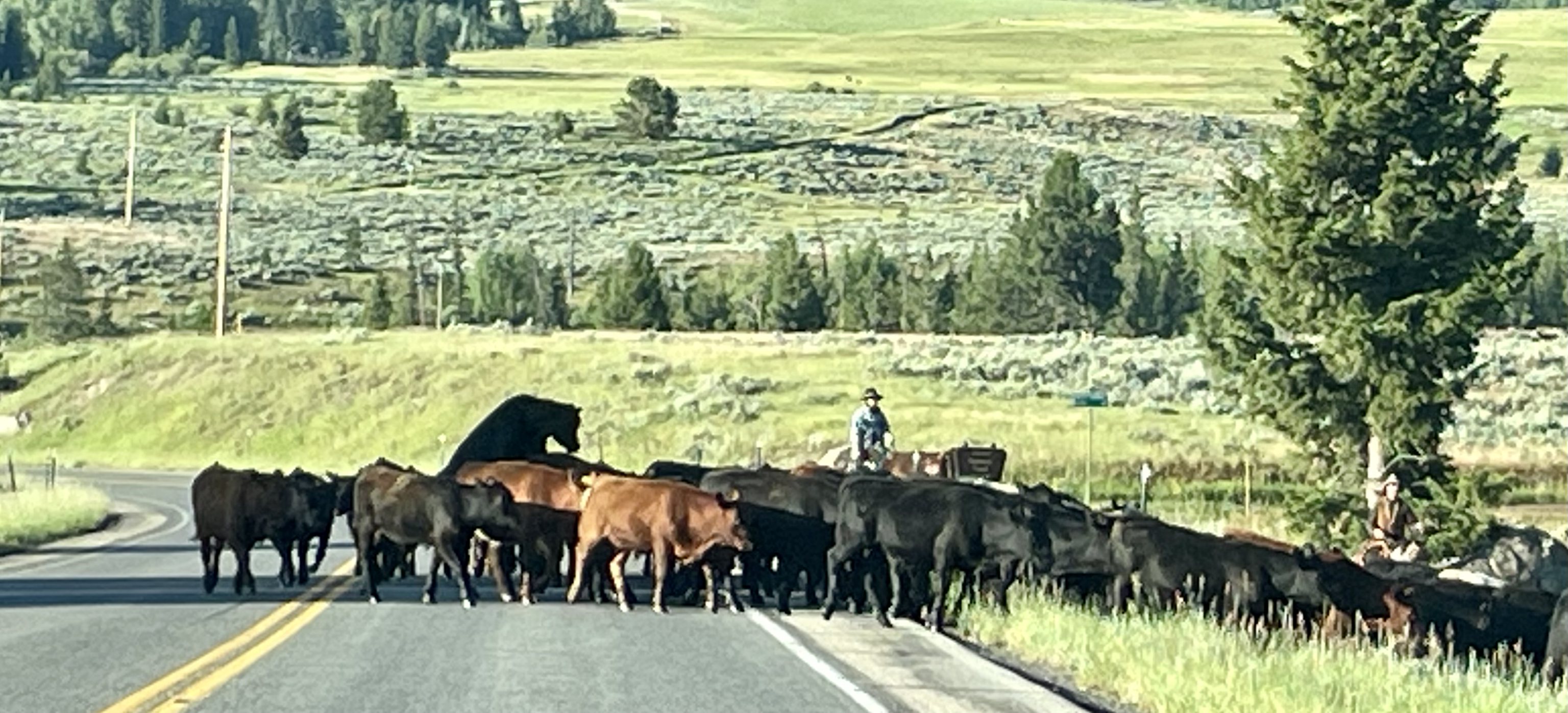In this vibrant, outdoor scene, a hilly field stretches into the background, covered with lush, dense, and thick greenery. Trees of varying sizes, including pine and evergreen, dot the landscape, contributing to the vivid greenery. A darker green patch of grass lies at the center with trees emerging from it, adding depth to the scenery. A telephone pole and a few electrical lines can be seen unobtrusively in the background. 

In the foreground, light green grass, some recently cut, forms a pasture, leading towards a two-lane highway. A herd of cattle, predominantly black with a few brown ones, is making its way across the road. The cattle appear to be heading towards the expansive field to graze. Among them is a noteworthy cow, seemingly more animated than the others. 

The scene includes a cowboy, dressed in blue with a smaller brimmed hat, mounted on a horse, shepherding the cattle across the highway. The solitary cedar-like tree standing tall against the soft light, alongside the long, rightward-cast shadows, suggests the photo was taken either in the early morning or late afternoon. The overall mix of elements lends a picturesque and possibly surreal quality to the image, making it momentarily difficult to ascertain its authenticity.